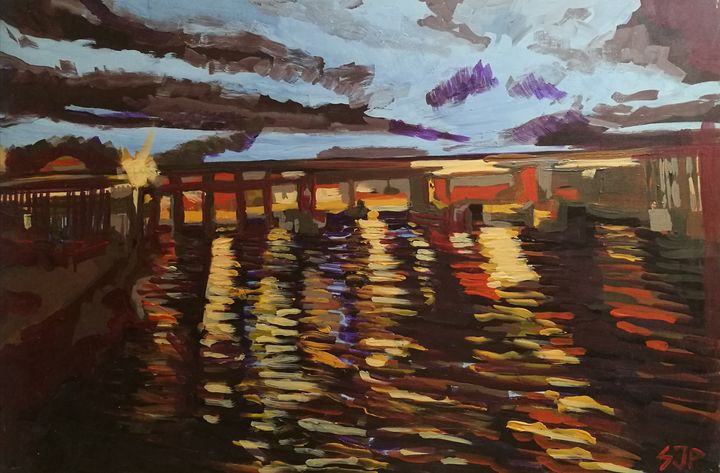This acrylic painting depicts a bridge at dusk under a dramatic sky filled with a mixture of blue, grey, purple, and dark clouds. The sky's complexity includes artistically interpreted, dreary clouds creating a moody atmosphere. The bridge, appearing arched and possibly wooden, spans across a dark, reflective river. The bridge is subtly outlined and shaded in tones of orange, white, cream, and yellow, casting a warm glow. Below, the water ripples softly, catching hues of yellow, blue, red, and gold, suggesting a light source to the right. To the left, a silhouetted structure resembling a coliseum appears, with a hint of a fiery glow nearby. The painting exudes an impressionistic style, emphasizing color and atmosphere over precise detail. Signed by the artist with "SJP" at the bottom, this scene beautifully captures the tranquil yet enigmatic interplay of light and shadow at dusk.